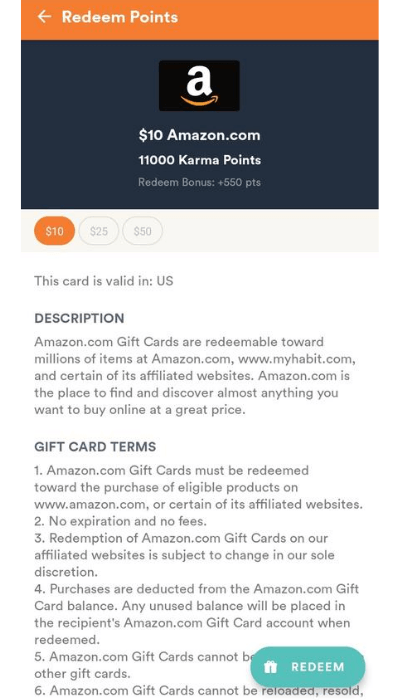A detailed screenshot for redeeming points for an Amazon gift card:
The image features a layout for redeeming points on a platform. At the very top, there is a prominent orange bar with white text that reads "Redeem Points." Beneath this, there is the iconic Amazon logo— a white "A" with a smile underneath—set on a black background. This black field is bordered by a blue area that provides additional information.

Within this blue area, text indicates options for redeeming a $10 Amazon gift card in exchange for 11,000 Karma points, with a bonus of 550 points. Below this, there are selectable options for $10, $25, and $50 denominations. The $10 option is highlighted and selected, prominently displayed in an orange capsule.

Further details describe the terms and usages of the gift card:
- This card is valid in the U.S.
- The description emphasizes that Amazon.com gift cards are redeemable towards millions of items on Amazon, MyHabit.com, and other affiliated websites.
- Amazon.com is noted as a place where you can find almost anything at a great price.

The gift card terms are meticulously listed:
1. The card must be redeemed towards available products.
2. There are no expiration dates or fees associated with the card.
3. Redemption on affiliated websites is subject to change.
4. Purchases will be deducted from the gift card balance.
5. Any unused balance will be applied to the gift card account and can be redeemed later.
6. The card cannot be combined with other gift cards, nor can it be reloaded or resold.

At the lower right-hand corner of the image, there is a sky-blue or teal-colored capsule button featuring a gift box icon. This button is labeled "Redeem" and partially overlaps the text detailing the gift card terms.